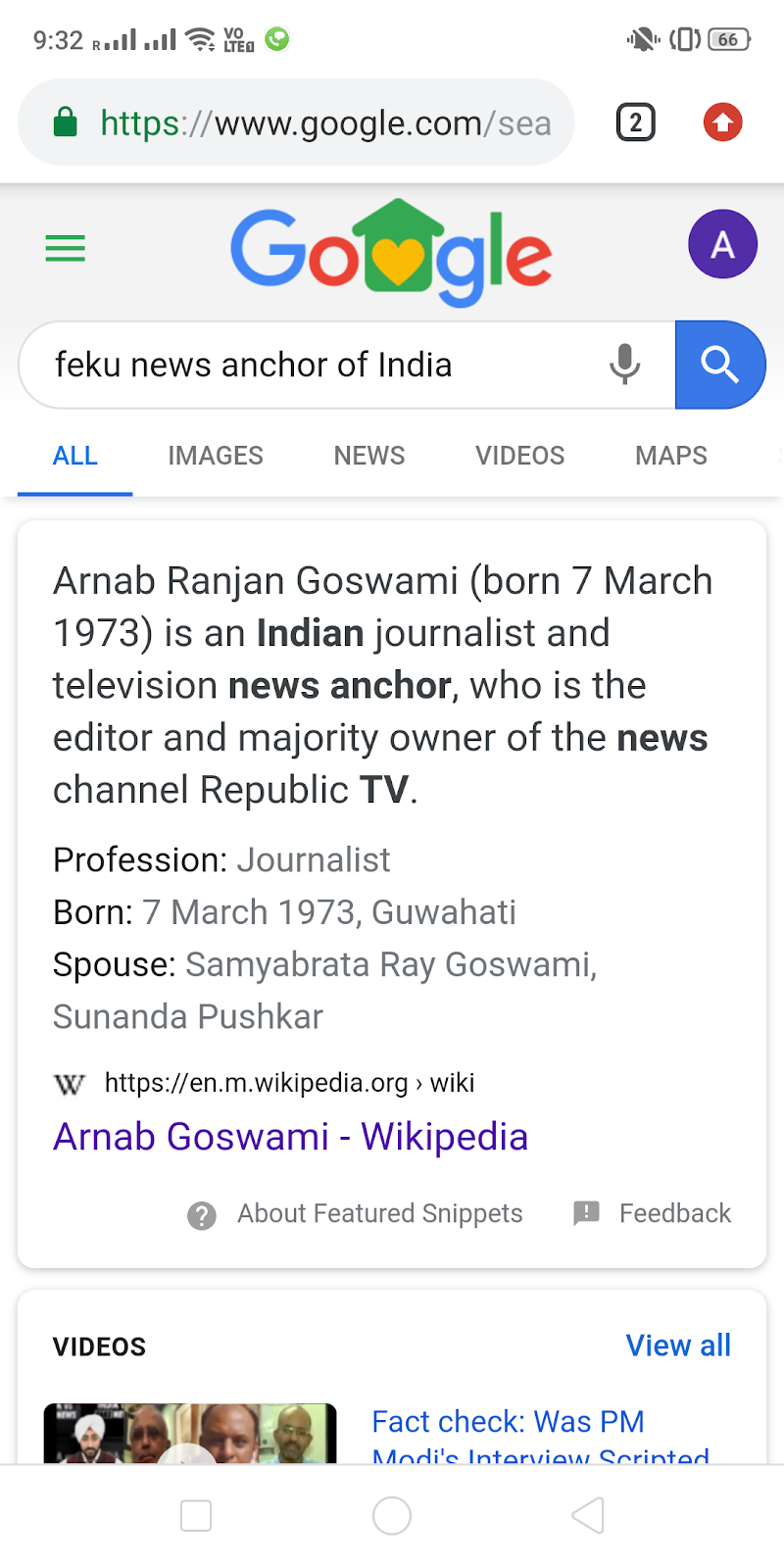A screenshot of a mobile Google search results page captured at 9:32 AM. The top left corner displays various phone icons, settings, and varying signal strengths, while the top right shows a battery level of 66%. The screen showcases the Google homepage with the search query "Feku News, anchor of India". The interface features the standard Google layout with a white background, subtle gray accents, and the iconic multi-colored (blue, red, green, yellow) Google logo. The search bar includes a blue button with a white magnifying glass icon.

Below the search bar, there are tabs for "All," "Images," "News," "Videos," and "Maps." The top search result under the "All" category is a Wikipedia entry for Arnab Ranjan Goswami, an Indian journalist, and television news anchor born on March 7, 1973, in Guwahati. The entry details his role as the editor and majority owner of Republic TV. Additional personal information includes his profession, birthdate, and spouse names: Samyabrata Ray Goswami and Sundar Pushkar, though it is unclear if one might be a former spouse. A link to the full Wikipedia article is provided. The screenshot also partially shows another section below, featuring video links, one of which is cut off at the bottom of the screen.